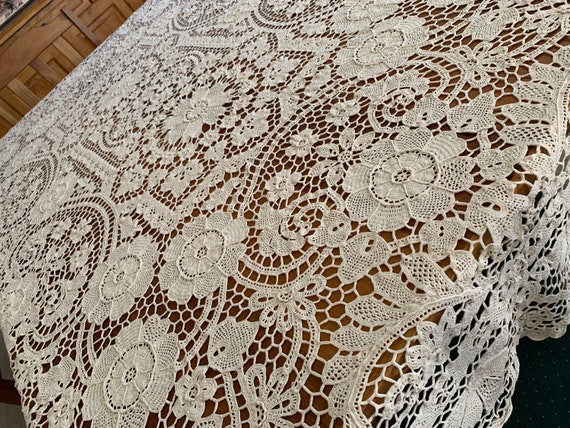This color photograph captures a top-down view of a dining scene, dominated by a large, white lace tablecloth adorned with intricate floral and leaf patterns. The tablecloth, with its heart-shaped petal designs and net-like mesh featuring large holes, allows glimpses of the rich brown wooden table underneath. The lace extends over the table's edge, revealing a contrasting black floor. In the background, beautifully crafted wooden cabinets and a brown dining chair add a touch of warmth and elegance to the setting.